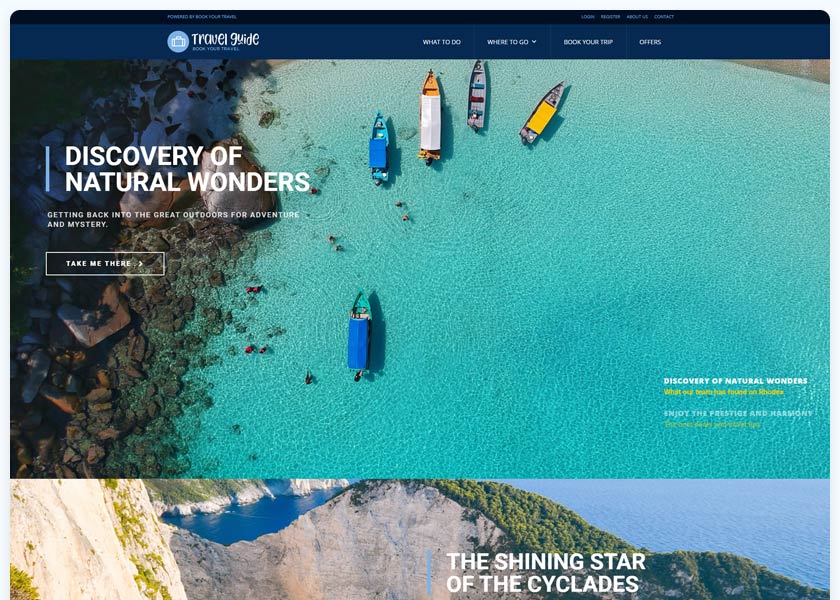The image portrays a dynamic travel guide website titled 'Travel Guide,' featuring various sections such as 'Book Your Travel,' 'What to Do,' 'Where to Go,' 'Book a Trip,' 'Offers,' 'Login,' and 'Register.' Central to the design is a prominent blue bar with white text proclaiming, 'Discovery of Natural Wonders.' It invites visitors to 'Come back into the great outdoors for adventure and mystery.'

The visual background showcases a stunning scene of clear blue waters with boats gliding over the surface. Surrounding the water are vibrant, colorful rock formations, possibly indicating a diverse and rich landscape. Further in the distance, you can see majestic mountains and dense forest greenery. A standout piece of text overlays this scenery, declaring 'The Shiniest Star,' suggesting that this location is a gem of natural beauty.

The overall layout is designed to inspire and inform users about the myriad of adventures awaiting them, blending picturesque visuals with engaging text to captivate the travel enthusiast's imagination.